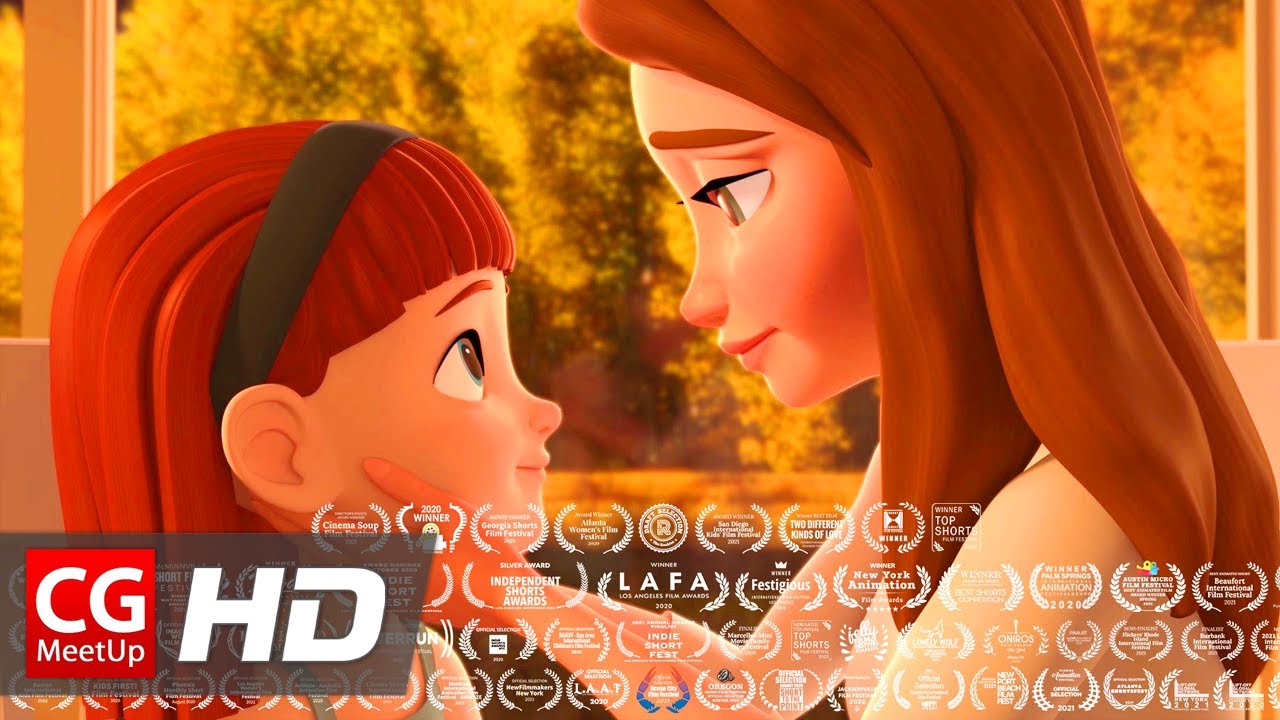This image is a detailed, computer-generated still shot from a short animated film. The scene captures an intimate moment between a mother and her daughter, emphasizing their close bond. The mother, who has long, medium brown hair with a hint of burnt orange, gently holds her daughter’s face in her hands, her green eyes reflecting a loving expression. The daughter, a small girl with red hair held back by a black headband, looks up at her mother with a soft, affectionate smile, her blue eyes mirroring her mother's gaze. They both are wearing simple attire; the little girl in a green tank top, standing in what appears to be an indoor setting with trees visible through a window in the background.

Beneath this touching scene, a black translucent banner displays numerous accolades in white text, showcasing the film's recognition at various festivals and competitions. Highlighted awards include "Winner Top Short Film," "LAFA Los Angeles Film Awards," "Fastidious New York Animation Award," among others. Additionally, a red and white symbol indicating "CG Meetup HD" is prominently featured, further marking the accolades’ significance. The overall color palette of the image is rich with reds, oranges, and yellows, adding warmth to the heartfelt moment.